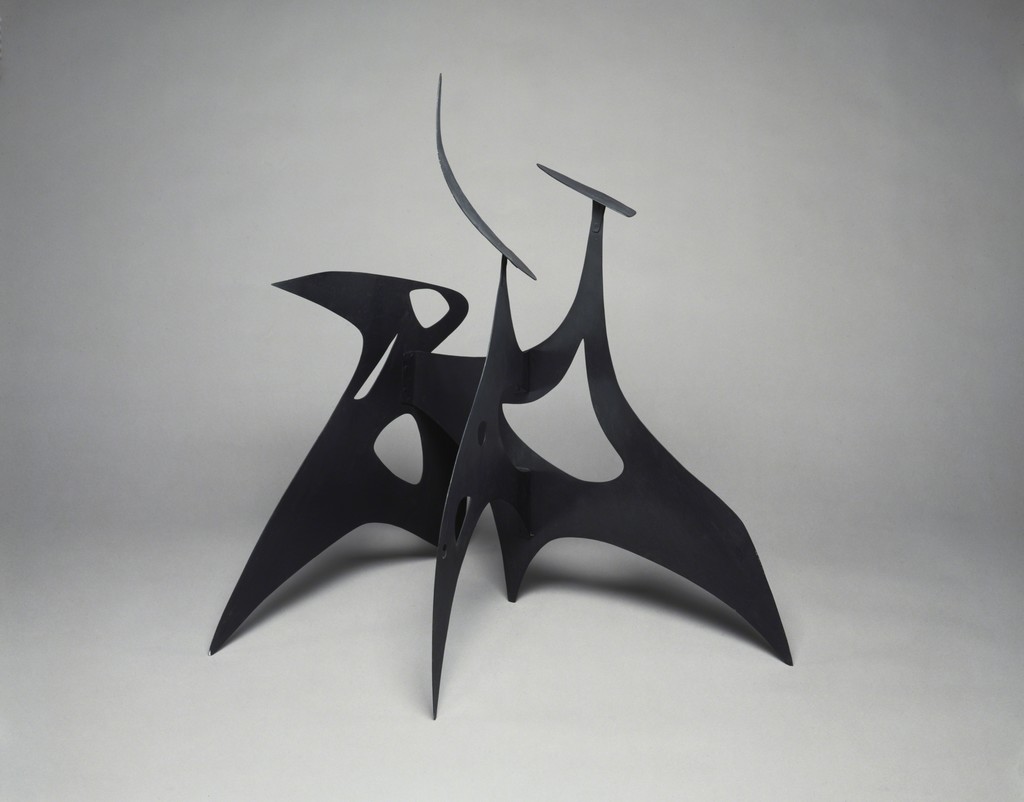The image depicts an abstract, black metal sculpture composed of three distinct, evenly spaced panels that converge toward the center. Positioned against a neutral gray background, the sculpture's construction reveals meticulous craftsmanship, featuring wavy, blade-like sheets of metal with various cutouts and curves. The left panel showcases two triangular openings, one at the top and another in the middle. The central panel is distinguished by a slender metallic element protruding from its upper section. On the rightmost panel, a prominent dome with a triangular cone-shaped cutout adds to the complexity of the composition. Additionally, each panel integrates sharp, spiky extensions—four legs spreading outward and two interior legs—all contributing to the sculpture's dynamic and intricate design.